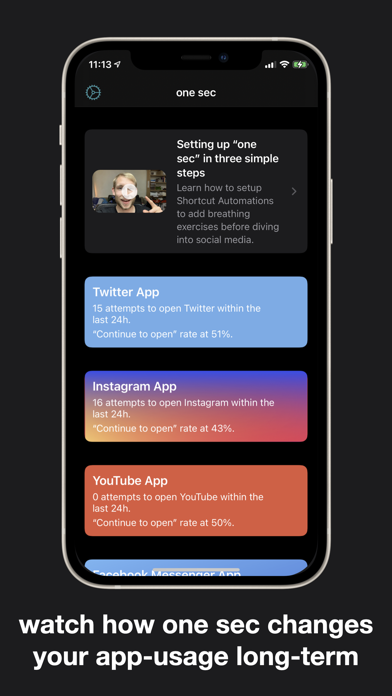This image captures a screenshot taken from a cell phone. The backdrop is entirely black, accentuating the details on the screen. 

At the top of the phone display, the time is shown as 11:13, with a small paper airplane icon indicating airplane mode, and a battery icon depicting that the device is currently charging and nearly full.

Towards the upper part of the screen, there is a teal circle with the text "1 sec SEC." Below this, a video prompt is visible, ready to be played, with the caption "Setting up 1 sec in 3 simple steps," followed by an explanatory paragraph.

As you scroll down on the screen, there is a sequence of app icons displayed: 
- A purple rectangle labeled "Twitter app."
- A rainbow-colored rectangle labeled "Instagram app."
- A red rectangle labeled "YouTube app."
- Lastly, a blue rectangle, partially cut off, indicating "Facebook Messenger app."

Just outside the phone screen at the bottom, crisp white text reads, "Watch how 1 sec changes your app usage long term."